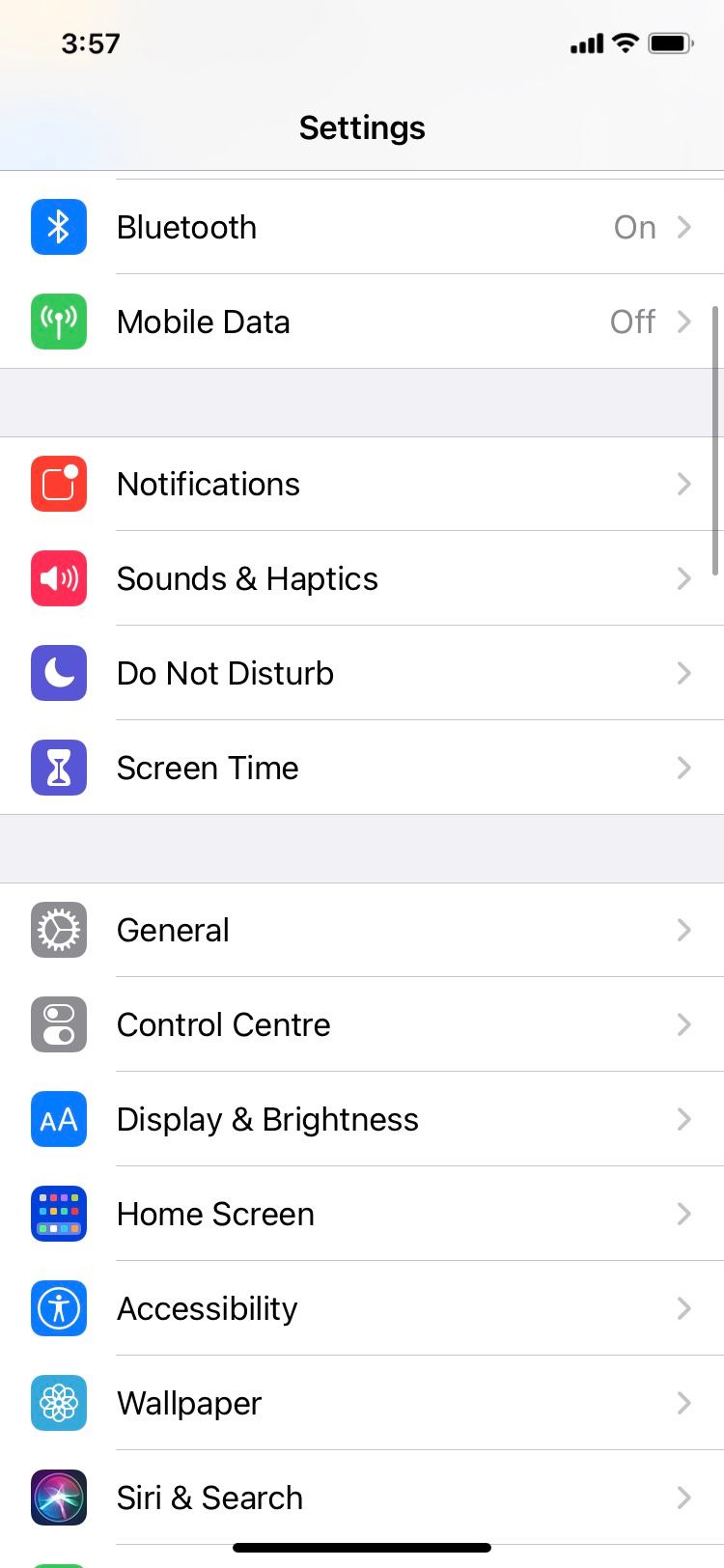This is a screenshot showcasing the settings menu on a smartphone. The image is a vertical white rectangular box. In the upper left corner, the time is prominently displayed in bold as "3:57". The upper right corner shows the Wi-Fi icon indicating full signal strength and a full battery icon. Below the status bar, the title "Settings" is centered at the top of the page. 

The menu is divided into sections by gray rectangular dividers. The first section includes:
1. **Bluetooth** - with the status "On" indicated in gray text and a right-facing arrow.
2. **Mobile Data** - with the status "Off" indicated in gray text and a right-facing arrow.

The next section, separated by a gray box, lists:
1. **Notifications**
2. **Sounds & Haptics**
3. **Do Not Disturb**
4. **Screen Time**

All items above have a right-facing arrow on their right side but no status indicators.

The final section, also separated by a gray box, includes:
1. **General**
2. **Control Center**
3. **Display & Brightness**
4. **Home Screen**
5. **Accessibility**
6. **Wallpaper**
7. **Siri & Search**

Each of these items also features a right-facing arrow on the right side, without status indicators.